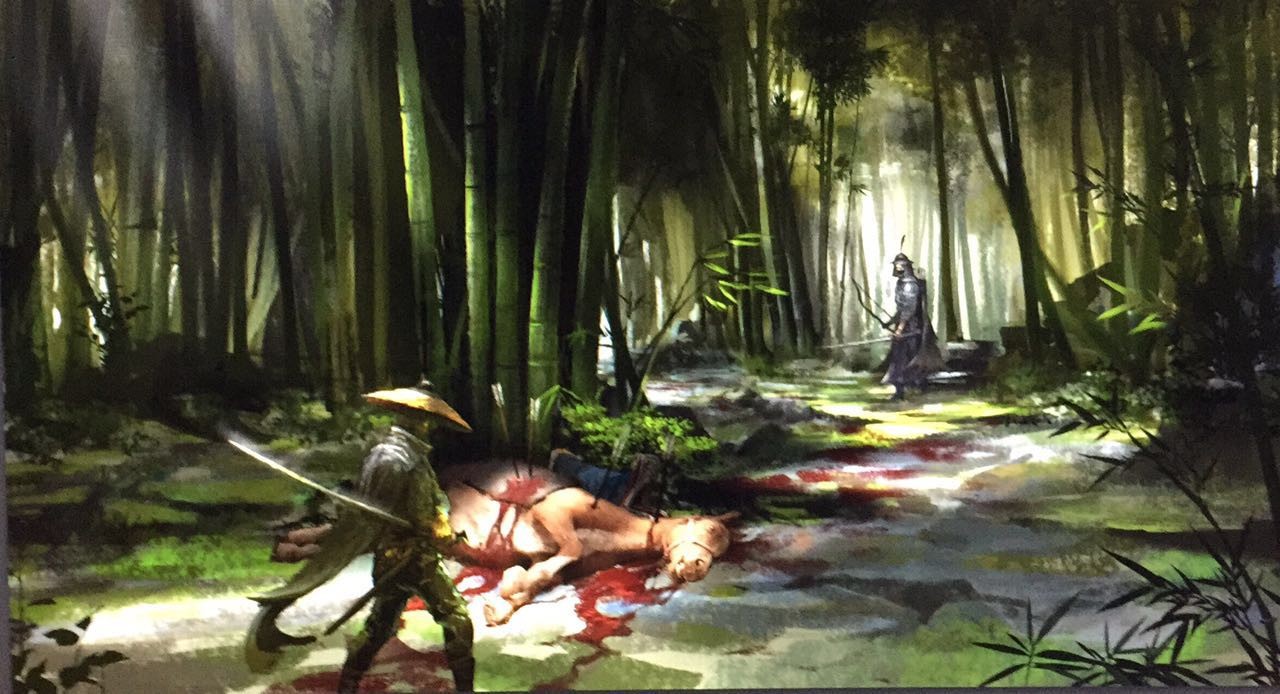This detailed illustration, possibly created using watercolors, depicts a dramatic scene set in a dark, dense bamboo forest with scarce sunlight filtering through. In the foreground, an injured horse lies bleeding on the ground, pierced by multiple arrows. Nearby stands a samurai warrior dressed in green, wearing a flat, tan straw hat, and holding a samurai sword poised behind his back, ready for combat. In the background, his adversary, clad in black samurai armor and armed with a bow and arrow, prepares for battle. The image captures the tense and somber moment before the clash, emphasizing the contrast between the ominous enemy and the resolute hero, set against the backdrop of an intricate and foreboding natural environment.